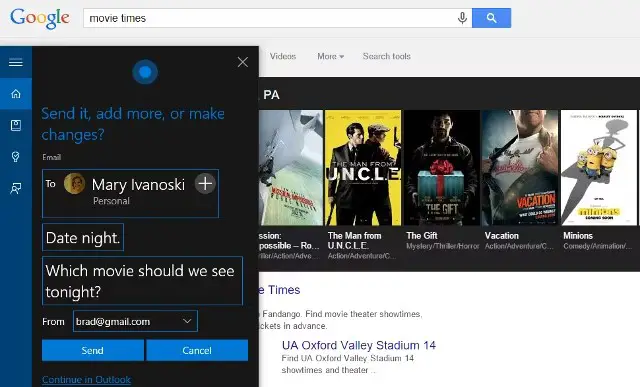A screenshot of a Google Movies interface for date night planning. The interface features a prominent black box with a blue vertical stripe and a blue border along the bottom, containing options to "Send it," "Add more," or "Make changes." The box is titled "Date Night: Which movie should we see tonight?" and is addressed to Mary Ivanski, from Brad (brad@gmail.com).

Beneath this, there's a "UA Oxford Valley Stadium 14 - Showtimes and Theater" section displaying a selection of movies currently showing, including "The Man from U.N.C.L.E.," "The Gift," "Vacation," and "Minions." The user-friendly interface suggests that selecting a movie for the date should be an uncomplicated process. The design is straightforward, facilitating easy navigation and movie selection.